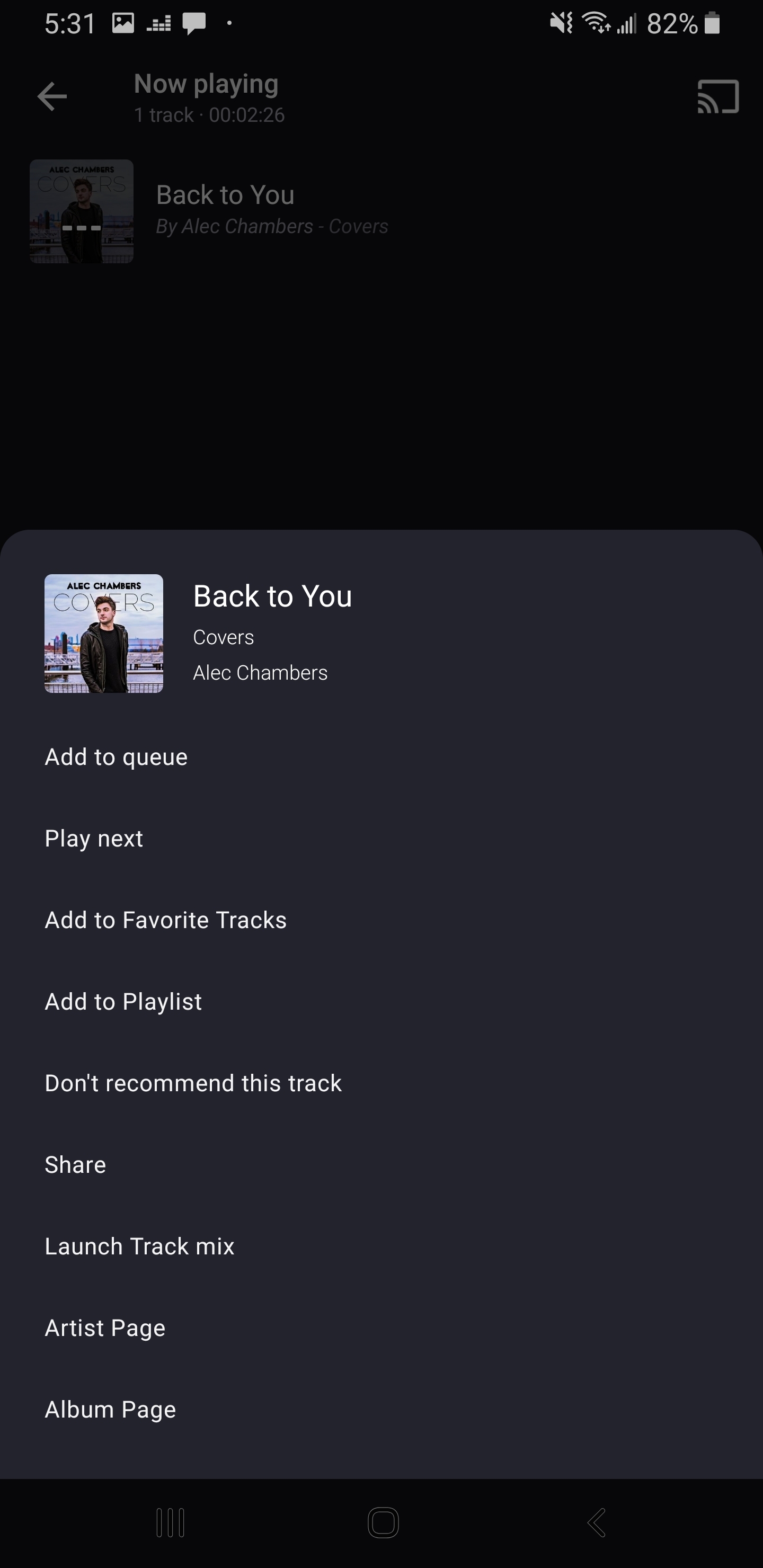The image showcases a smartphone screen displaying a music playlist. At the top-left corner, the time is 5:31, accompanied by icons for various apps including Photos, Music, and Messaging. The top-right corner features additional phone status icons such as the "no sound" icon, Wi-Fi signal, network signal, and a battery icon indicating 82% charge. Below these, in a grayed-out section, there is a currently playing track: "Back to You," a 2-minute and 26-second cover by Alec Chambers from his album "Covers." At the bottom of the screen, there is a prominent, non-grayed-out box that details the process for adding the track to the playlist.